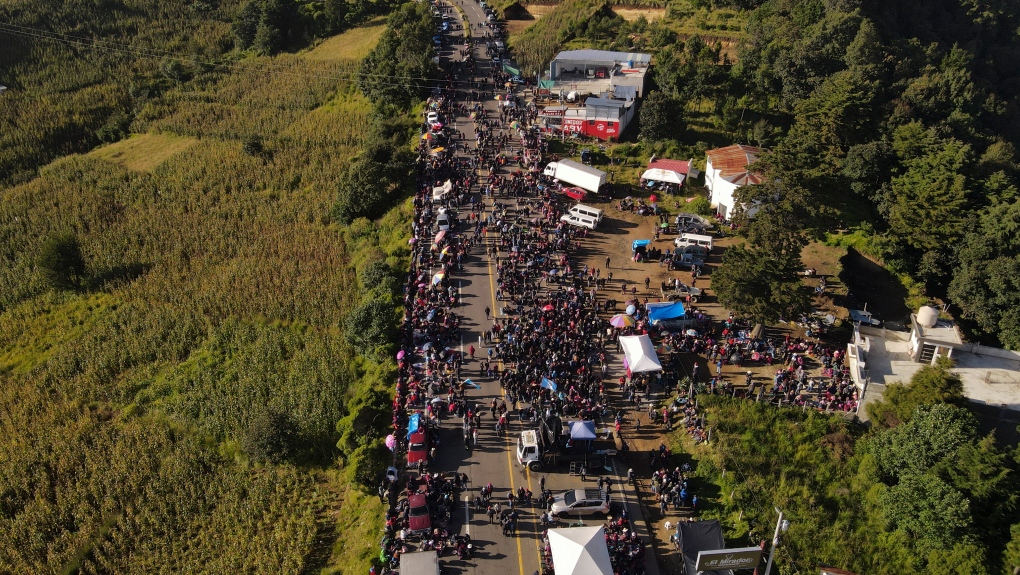This detailed aerial photograph, taken under a bright sunlit sky, captures a large and vibrant gathering of people on a wide street in a setting that resembles a bustling outdoor market or festival. Encompassed by lush green trees—darker and denser on the right side—the street is filled with hundreds of people, creating a lively and colorful scene. Numerous vehicles, including two red cars on the lower right side, a flatbed truck, and a white truck in the background, line the street. The image reveals various structures set up for the event: vendors with umbrellas and tents, contributing to the festive atmosphere. To the right, three prominent buildings are visible—the topmost is red and square, the middle one is rounded with an orange roof, and the bottom one is tan and cement-like. Additionally, a white building and a silo can be seen further to the right in this semi-rural, farmland-like location. The photograph richly conveys the joy and busyness of the event with intricate details of both the people and their surroundings.